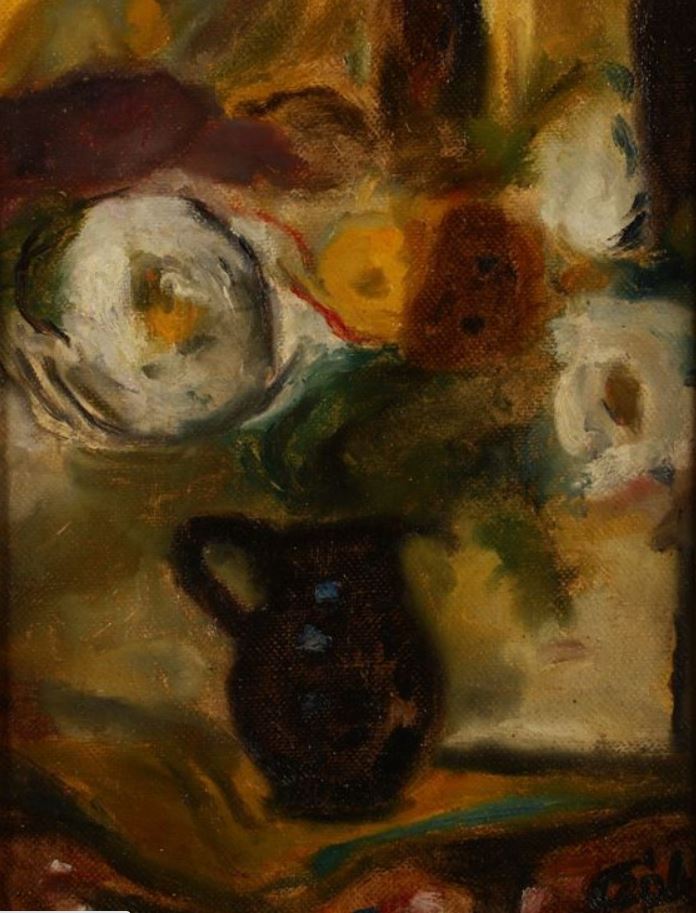This blurry and unfocused rectangular art image, approximately six inches tall and three inches wide, features a dark brown vase or jug with a handle on the left and a cupped lip on the right, positioned at the center bottom. The vase holds an assortment of flowers, with distinct shades including white with yellow centers, orange, burgundy, and pink. Several green stems and leaves are intertwined among the flowers. Surrounding the central arrangement are swirls and blotches of various colors: greens, browns, yellows, and oranges, creating a harmonious yet indistinct backdrop. The base of the painting shows the vase seemingly resting on a blurred, multicolored platform, with hints of red and a green stripe. The overall tones of the painting blend together with no clear outlines, inviting viewers to let their eyes adjust to appreciate the beauty of the abstract composition.